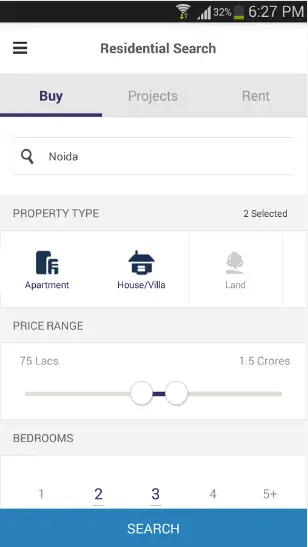A screenshot from an Android phone displaying a residential search app interface is depicted. At the very top, the standard black Android status bar exhibits various icons on the right, including the Wi-Fi signal, mobile data indicator, battery level at 32%, and the time reading 6:27 PM.

Beneath the status bar, the app's header is labeled "Residential Search." On the left side of this header, there's a three-line menu icon, signaling additional options or settings. Directly below this, a gray navigation bar offers options for "Buy," "Projects," and "Rent," with "Buy" highlighted in blue, indicating the current active selection.

A search bar situated below the navigation bar contains a magnifying glass icon and the text "Noida," specifying the search location. Moving further down, there's a section for selecting the property type, where two options— "Apartment" and "House/Villa"—are highlighted in blue, while "Land" remains gray, indicating it is not selected.

The next section presents a price range selector, depicted as a sliding scale with adjustable limits ranging from "75 Lakhs" to "1.5 Crores." Below the price range selector, a set of bedroom options from "1" through "5+" is displayed. Here, the numbers "2" and "3" are highlighted in blue, suggesting the user's preferred choices.

At the very bottom of the screen, a prominent blue "Search" button is positioned, ready to initiate the search with the specified criteria. Overall, the image shows a detailed and specific setup for finding a residential property within a designated area and parameter set.